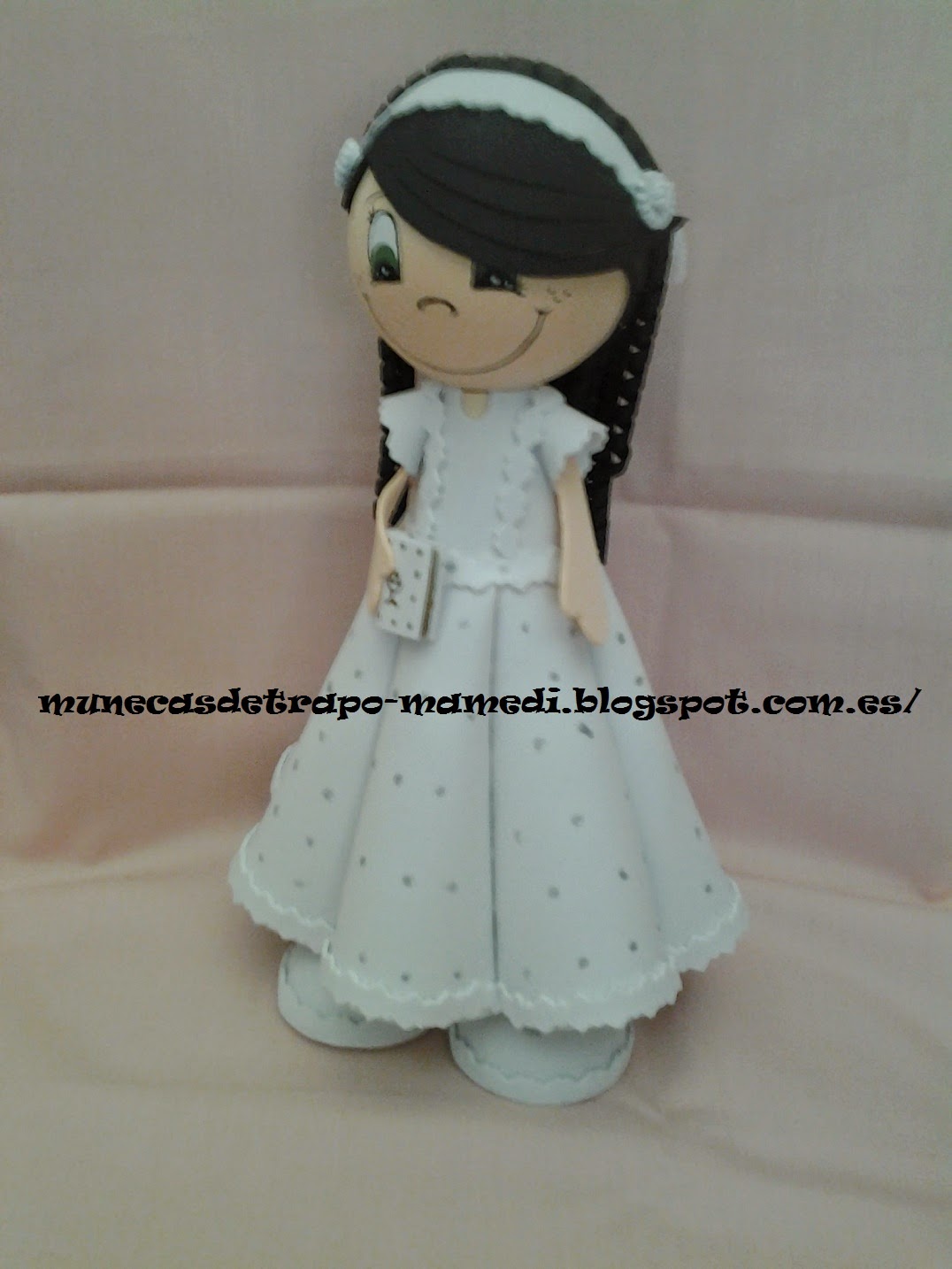This image features a highly stylized doll with a disproportionately large spherical head and wide, expressive features. The doll has enormous eyes that take up almost half of its face, a small arched nose, and a large, wide smile. She wears a white short-sleeve dress adorned with polka dots on the skirt area and decorated with lace trim. The material of the doll appears to be rubber-like. Her straight, long black hair, which includes bangs swooping over one side of her face, is topped with a white headband. The doll holds a small white book in her right hand. Positioned in what seems to be the corner of a couch, the background includes a bit of white fabric. Text across the image reads "municastetrapomamedy.blogspot.com.es slash," and the doll stands on giant white shoes, making her easy to set up or display.